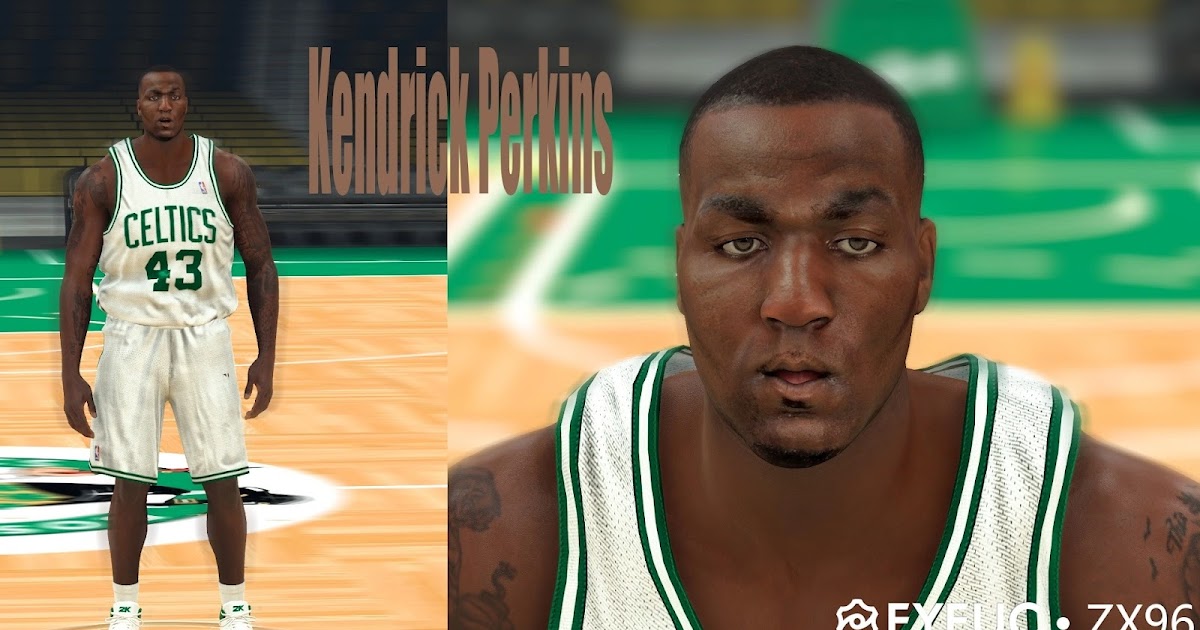The image comprises two photographs of a black man named Kendrick Perkins set against a basketball court backdrop. 

The photograph on the right features Perkins standing in his Celtics uniform, designated with the number 43, positioned on a polished basketball court. He stands confidently, showcasing his athletic physique.

The photograph on the left presents a closer view, capturing Perkins from the waist up, providing a clearer view of his facial features and tattoos adorning his arms. This close-up also retains the basketball court in the background but accentuates the details of his facial expressions and tattoos.

Between these images, the name "Kendrick Perkins" is prominently displayed in brown text. Additional elements include partial lettering in the lower left corner, which reads "E-X-E" followed by partially obscured characters and then "O" and ".7-X-9-6." In the background of the close-up image, there is a green patch and a yellow object extending to the right. Additionally, in the image of Perkins standing, there is a white circle with green details, possibly hinting at the Celtics logo, although it's not entirely clear.

This composition effectively highlights Kendrick Perkins, accentuating his identity and affiliation with the Celtics, while blending athletic and personal elements through tattoos and facial expressions.